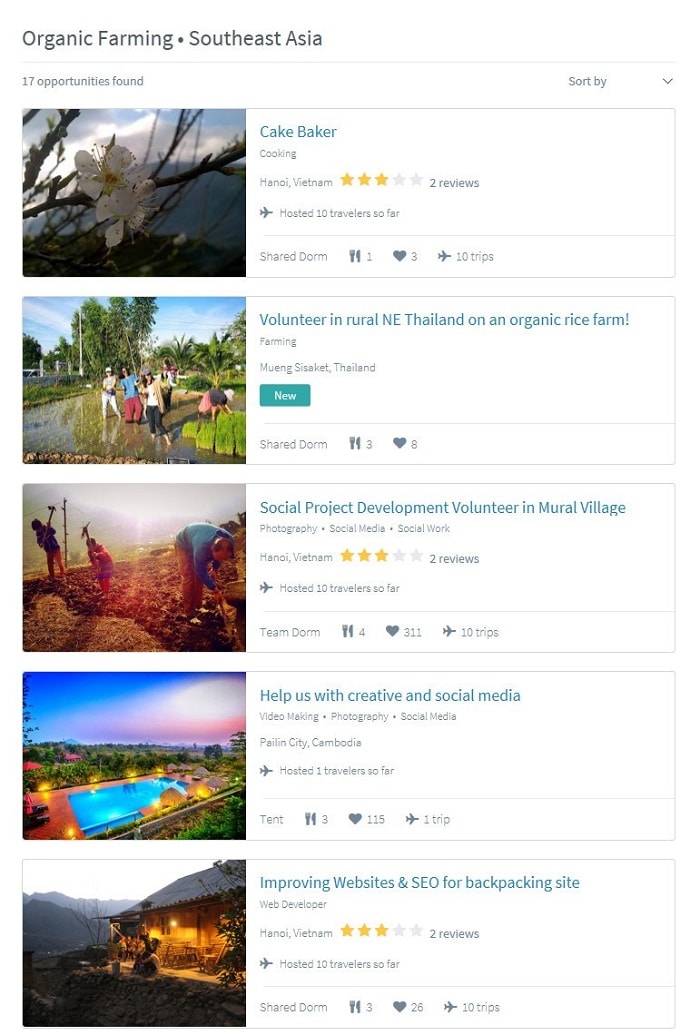This screenshot displays a search results page focused on organic farming opportunities in Southeast Asia, showing the first five of 17 total entries. Each listing includes a photograph on the left and some descriptive text on the right. 

At the top, there's an image of lush flora in a tree with the title "Cake Baker" featuring only two reviews and a rating of three out of five stars. The next listing highlights a newly posted opportunity titled "Volunteer in rural Northeast Thailand on an organic rice farm."

Scrolling down further, there's a project labeled "Social Project Development," inviting volunteers to contribute to a mural village. Next, an opportunity titled "Help Us with Creative and Social Media" appears. 

The final visible listing, before requiring further scrolling, is "Improving Websites and SEO for a Backpacking Site," specifically targeting web developers. This entry, related to Hano, Vietnam, has a three-star rating from two reviews and notes that it has hosted 10 travelers so far. Various icons are visible at the bottom of each listing, presumably representing additional details or features offered by each opportunity.